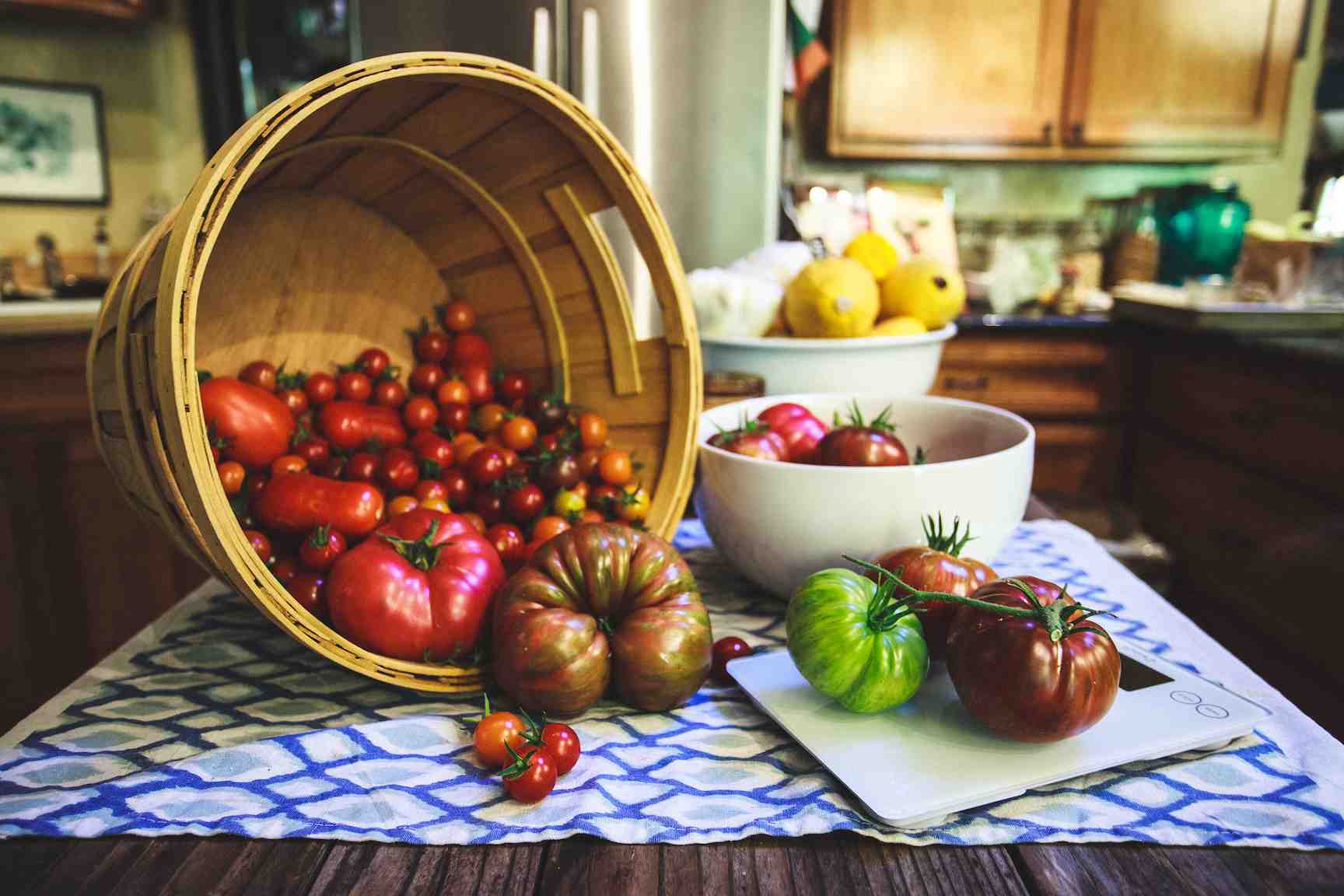This photograph captures a vibrant kitchen scene with a wooden table at its center, draped in a blue and white tablecloth. The central highlight is a large wicker basket tipped over, spilling an array of tomatoes across the table. The basket overflows with a variety of cherry, Roma, beefsteak, and heirloom tomatoes displaying a spectrum of colors from green to red to dark purple. At the forefront, three uniquely shaped heirloom tomatoes—one green, one dark magenta, and one orangish red—are scattered. To the right corner, a white bowl brims with more tomatoes, adding to the bountiful display. Behind this, another white bowl filled with bright yellow lemons offers a striking contrast. The surrounding kitchen features wooden cabinets, a silver-doored refrigerator, and countertops in the background, adorned with additional details like a wall picture above the counter. The overall composition emphasizes the rich, colorful harvest of tomatoes set against the warm, homely backdrop of a kitchen.